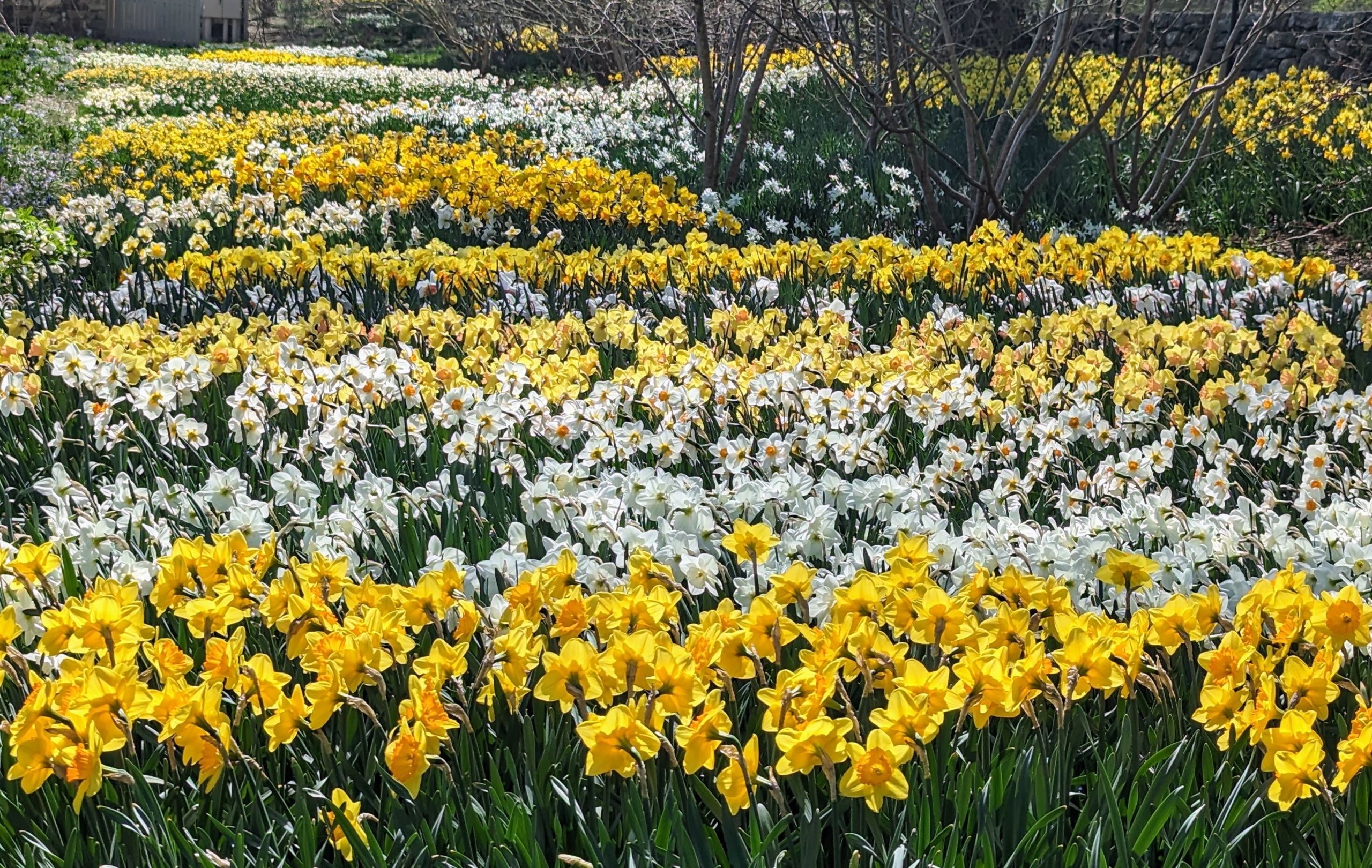The photograph captures an outdoor landscape filled with meticulously arranged rows of vibrant flowers, extending into the distance. The foreground features an array of yellow flowers with long green stems and narrow leaves, each bloom boasting six petals and a darker yellow center. Alternating rows of white and yellow flowers with yellow centers stretch horizontally across the image, creating a striking pattern that continues up to the middle. Along the top right quadrant, there are a few small, leafless trees with thin branches, while in the upper left corner, a glimpse of a gray building, possibly a shed with an open garage door, can be seen. The scene is bathed in natural light, emphasizing the beauty and structure of the flower rows set against the simple backdrop of bare trees and a distant building.